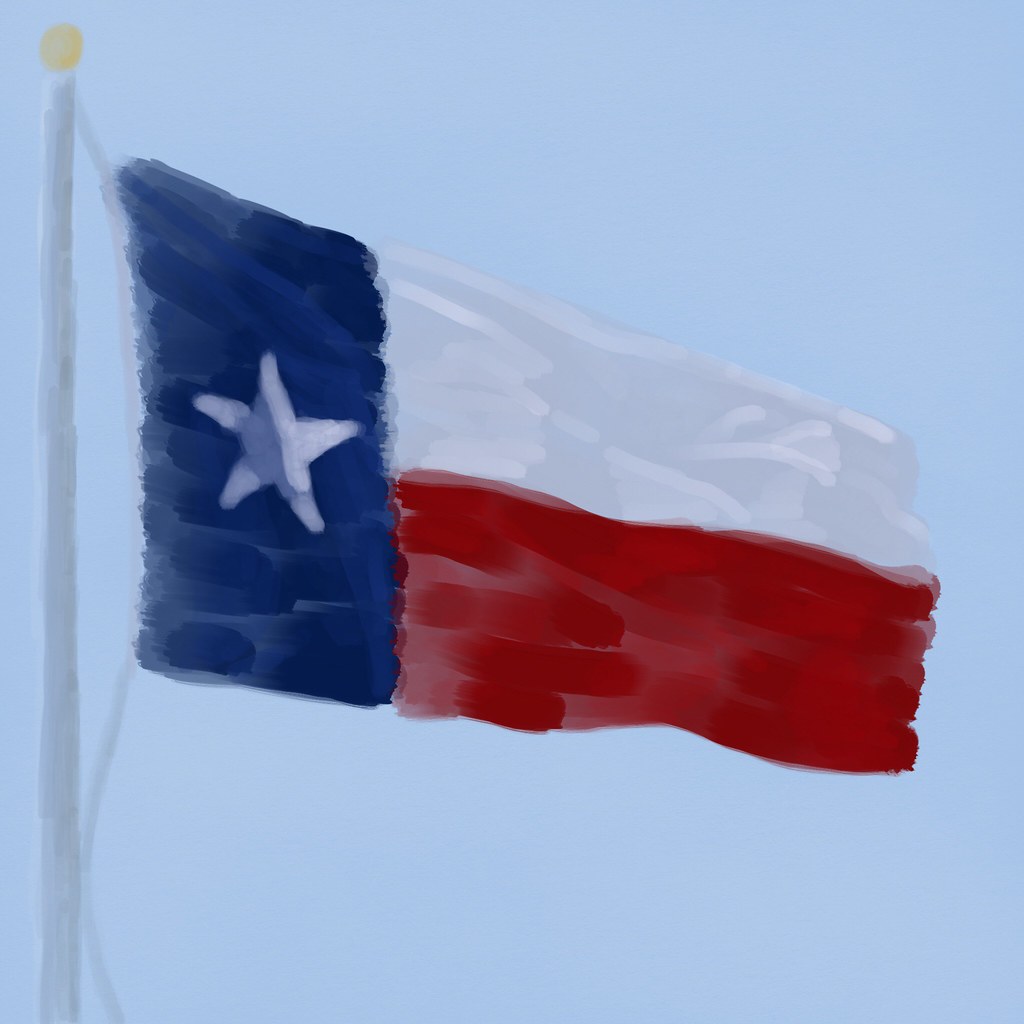The painting depicts a close-up view of the Texas state flag waving on a flagpole, set against a light blue background that suggests the sky. On the left side of the image is a thick silver or gray pole with a gold ball finial at the top. A gray rope runs from the gold ball down off the frame, suspending the flag. The flag itself features a vertical blue field with a white star near the pole, and horizontal stripes—white at the top and red at the bottom—extending to the right. The flag appears to be fluttering in the wind, and the artist’s painterly style is evident in the visible brushstrokes that give texture to the colors. This evocative use of watercolor accentuates the dynamic, waving motion of the flag, symbolizing the Lone Star State, Texas.